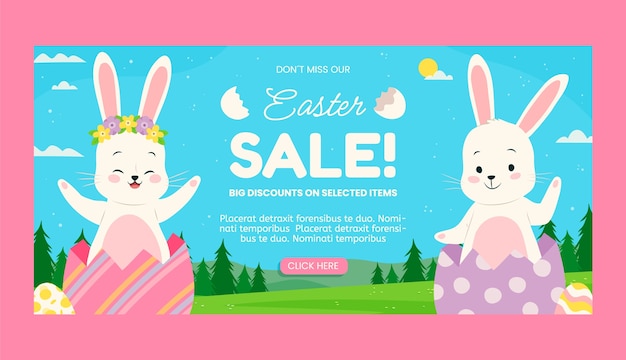The image depicts a vibrant Easter-themed promotional advertisement. The entire ad is framed by a pink border. At the top center of the image, the text reads "Don't miss our," while further down, in the middle, it says "Easter sale," with "Easter" elegantly written in cursive and "sale" boldly displayed in large white text. The phrase "big discounts on selected items" appears beneath the word "sale."

To the left and right of the word "Easter," there are illustrations of cracked eggshells symbolizing the festive theme. At the very bottom middle of the image, the words "click here" are prominently featured in white text on a pink oval background.

Adding to the cheerful display, there are cartoon bunnies on both sides of the text. The bunny on the right is white and peeks out from a purple eggshell adorned with white dots. The bunny on the left, also white, sports a floral headband with yellow and purple flowers and is inside a pastel pink egg decorated with blue, light pink, and yellow stripes.

The background of the image features a blue sky, complemented by lush green trees at the bottom, enhancing the springtime ambiance of the advertisement.